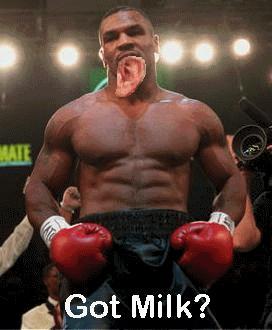The image is a meme featuring a topless black male boxer resembling Mike Tyson, wearing black shorts and red boxing gloves with white wristbands. He stands with his fists clenched in front of his body. Notably, an enlarged human ear appears to be hanging from his mouth, suggestive of a photoshopped addition. In the background, spotlights form a blurred row of white orbs across the top, creating a dramatic effect. On the bottom left, the partial view of people's raised hands can be seen, along with a person standing behind the boxer. To the right side, there is a visible camera. Imposed in white text across the image is the phrase "Got Milk?" with a question mark. Additionally, part of the text "M-A-T-E" in yellow letters is discernible on the middle left side of the image.